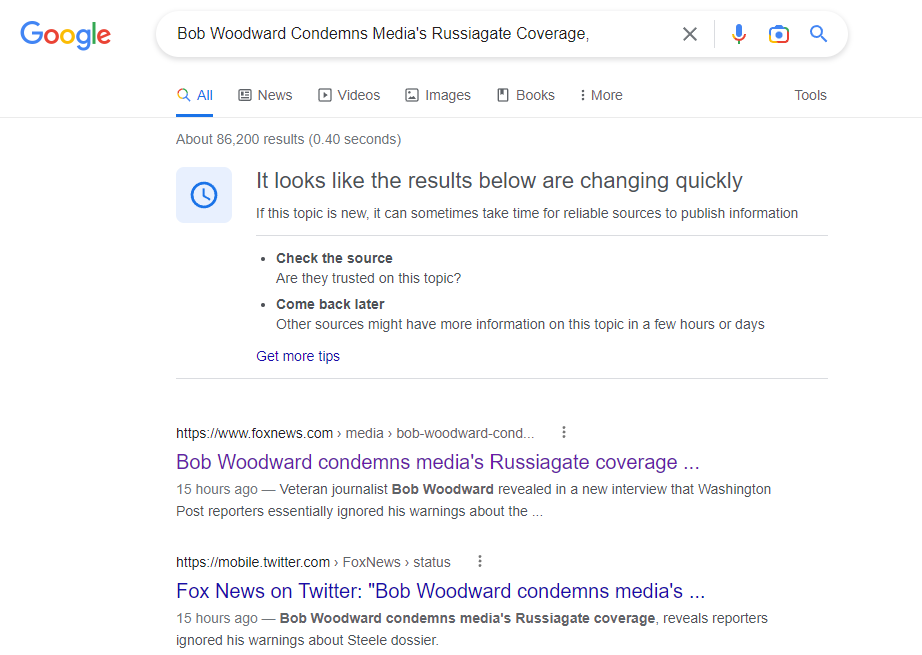This image captures a Google search results page displaying scrutiny over the media's coverage of Russiagate. At the top, the iconic Google logo appears in its traditional colors: blue, red, yellow, and green, followed by a blue underline. Below the logo, the search bar contains the query “Bob Woodward condemns media's Russiagate coverage,” with icons for microphone, camera, and search functionality flanking it.

To the right of the search bar, various search categories are listed in black, including 'All,' 'News,' 'Videos,' 'Images,' 'Books,' with an additional "Tools" option on the far right. A search results count of approximately 86,200, achieved in 0.40 seconds, is displayed underneath these options.

Prominently, a blue box with a clock icon warns: "It looks like the results below are changing quickly." This message is followed by a caution: "If this topic is new, it can sometimes take time for reliable sources to publish information," and an advisory in bold: "Check the source and come back later."

Further down, the first search result, highlighted in purple, links to a foxnews.com article titled "Bob Woodward condemns media Russiagate coverage," posted 15 hours ago. Beneath this, a snippet from Fox News' Twitter reiterates the condemnation, also posted 15 hours ago, with an accompanying explanation.